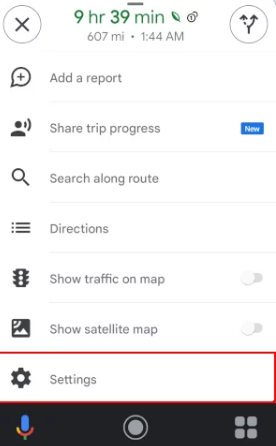The image depicts a smartphone screen displaying a navigation application in vertical orientation. The top of the screen shows a travel duration of "9 hours 39 minutes" in green text, with the distance listed as "607 miles" and the time "1:44 AM." There is an "X" inside a circle on the left side.

Below this information, a circular icon resembling a "Y" with upward arrows on either side and the label "Add a report" are visible. The next section includes "Share trip progress," accompanied by a blue bar labeled "NEW" on the right side. Following this, "Search along route" and "Directions" are listed, each with corresponding gray icons on the left.

Further down, options to "Show traffic on map" and "Show satellite map" are displayed. A red-outlined bar labeled "Settings" appears next. At the bottom of the screen, a black bar features a microphone icon, a home button, and a square box icon.